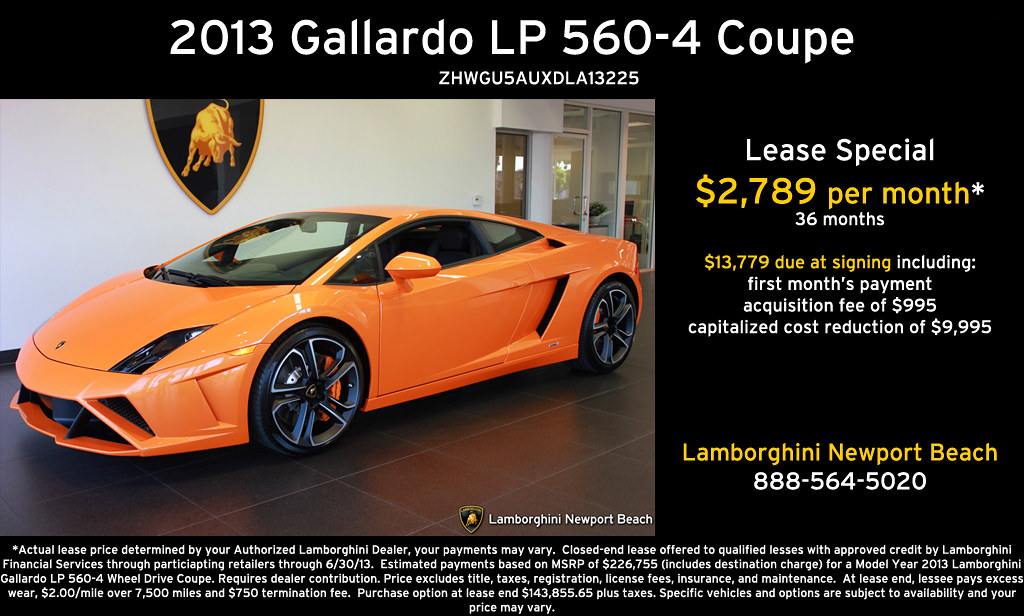This detailed promotional image highlights the lease offer for a 2013 Gallardo LP 560-4 Coupe, featuring an orange two-door Lamborghini with black rims parked inside a sleek dealership showroom. The background of the ad is black, providing a sharp contrast to emphasize the vehicle and text details. The upper part of the image, in white lettering, states "2013 Gallardo LP 560-4 Coupe" along with the code ZHWGU5AUXDLA13225. On the left side, nearly half of the image is occupied by the striking photo of the sports car, with an eye-catching gold bull Lamborghini logo on a poster against the white wall behind it. 

On the right, the ad details the Lease Special in white and yellow text: "$2,789 per month, 36 months, $13,779 due at signing including first month's payment, an acquisition fee of $995, and a capitalized cost reduction of $9,995." Below these terms, it lists the dealership as "Lamborghini Newport Beach" in yellow, followed by the contact number "888-564-5020" in white. At the bottom, the card includes a paragraph of disclaimer text explaining the terms and conditions of the lease offer.